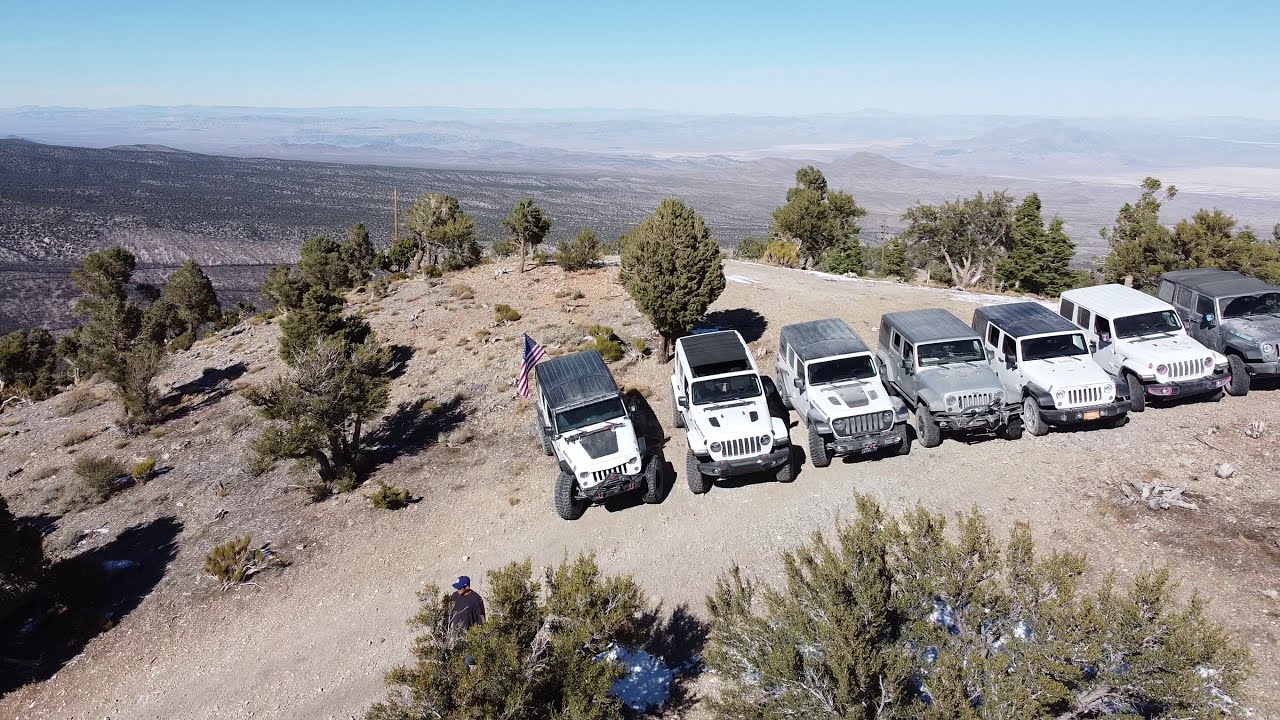The image depicts an elevated, desolate area reminiscent of a mesa or canyon, characterized by a mix of dirt, rocky terrain, and various types of trees and scrub pines scattered across the landscape. In the foreground, there's a line of seven Jeeps, predominantly in shades of white, gray, and black, with the one on the left displaying an American flag at the back. The Jeeps are parked facing the camera and look quite dirty. Among the few people present, a man can be seen standing near some bushes in the bottom middle left part of the image, wearing a dark gray shirt and a blue baseball cap. The background reveals a sweeping view of distant lands, shrouded in a slight haze, with a vast expanse of mountains stretching to the horizon under a mostly clear, sunny blue sky.